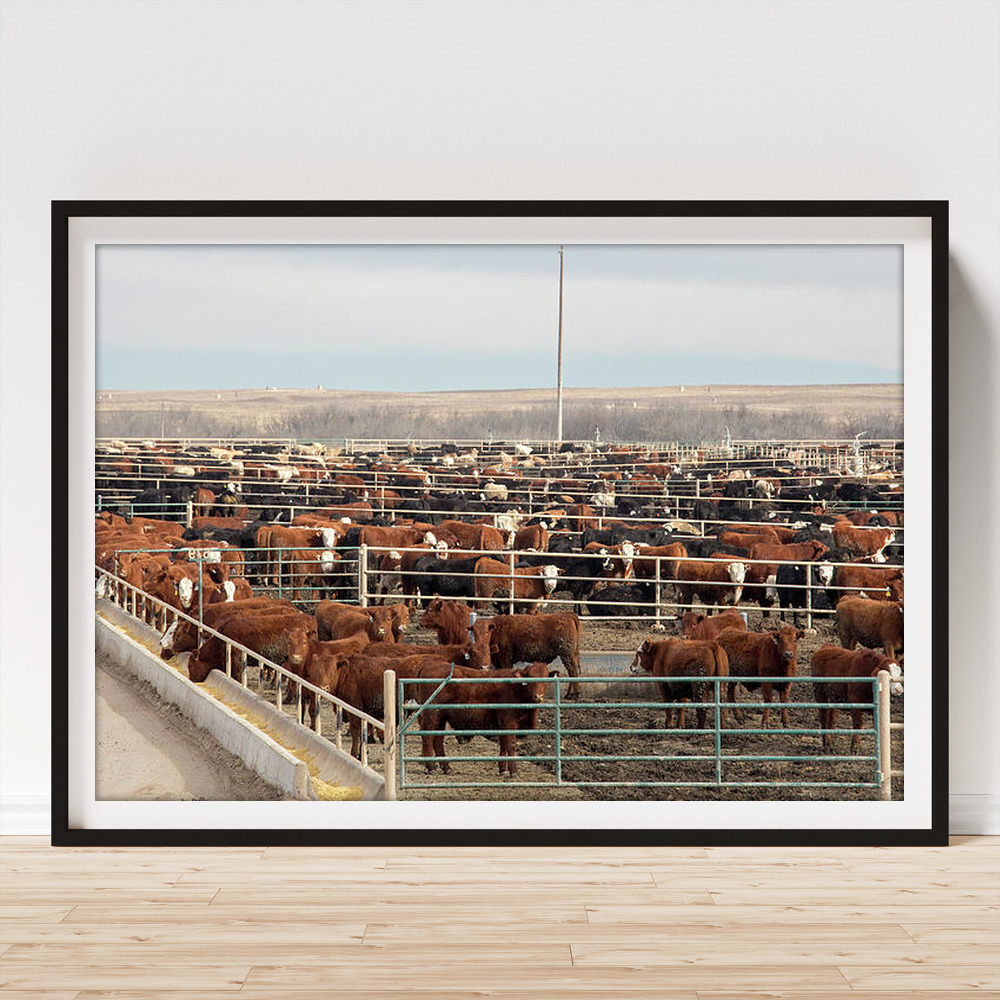The image depicts a photograph set in a black, thin frame with a white inner border. The photograph itself illustrates a farm scene filled with numerous cattle of varying colors, including browns, blacks, and some with white faces and ear tags. The cows are packed closely together within a gated area, which comprises silver metal fencing and white concrete barriers. The background reveals a dry, brown landscape with a blue sky and scattered white clouds above. The framed picture is positioned on a light wooden floor against a white wall, with visible white trim at the base, confirming that it rests on the floor.